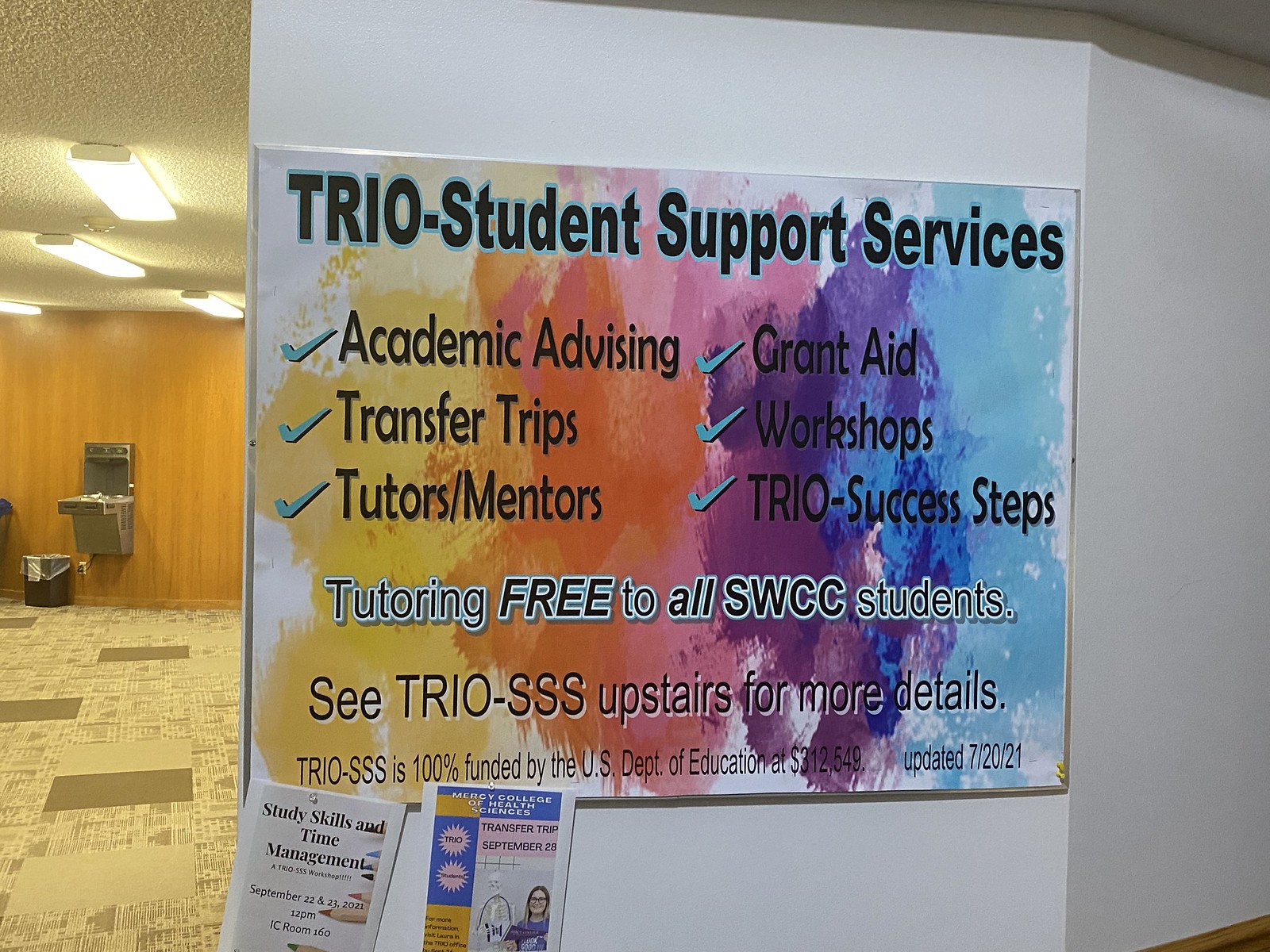The image is a wide rectangular photo of a vibrant sign attached to a white wall in an office building, possibly an educational institution. The sign reads "TRIO Student Support Services" at the top, followed by a list of services in black text, which includes Academic Advising, Transfer Trips, Tutors-Mentors, Grant Aid, Workshops, and TRIO Success Steps. Additionally, it mentions that Tutoring is free to all SWCC students, though it doesn't specify what SWCC stands for. The sign is colorfully designed with paint splatters that transition from yellow on the left to blue on the right, and it is framed by blue outlines. The background of the photo shows a light beige-greenish-brown carpeted room on the left, and an orangey-brown wall with a silver water fountain in the middle. The image captures ceiling lights and a hallway, emphasizing the office-like environment where the sign is prominently displayed for everyone to see.